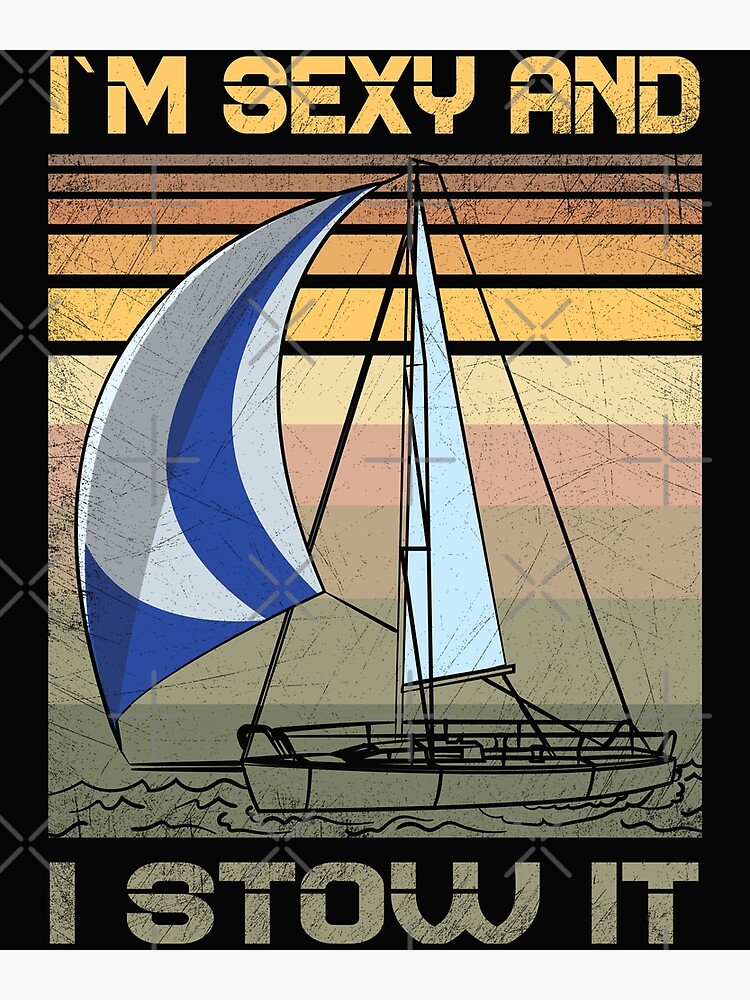This image features a retro-style poster with a humorous message. At the top, large capital letters in yellow spell out "I'M SEXY AND," and at the bottom, text in light green reads "I STOW IT," all set against a black background. Centered in the image is a small, simply drawn sailboat rendered in a combination of light gray and black. The main sail is striking with its stylized royal blue and white stripes, complemented by a smaller, narrower, almost white sail. Extending downward are ropes adding to the nautical theme. Behind the sailboat, the background is adorned with an array of horizontal stripes in varying widths and colors—from deep olive green at the bottom, through shades of brown, orange, pink, tan, yellow, to lighter and brighter hues as they progress upwards. These colorful bands create a nostalgic feel, emphasizing the playful and stylish nature of the poster. Additionally, subtle watermarks hint at copyright protection, suggesting this graphic is designed to deter unauthorized use.